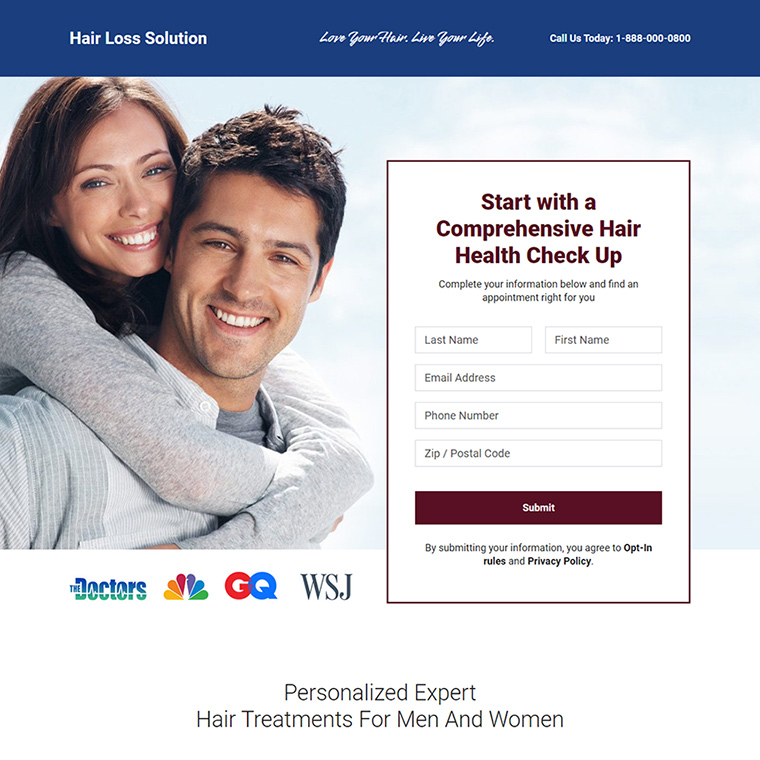Screenshot Description: Hair Loss Solution Advertisement

The screenshot features an advertisement for "Hair Loss Solution" with a visually appealing design. 

**Top Section**: 
- A vibrant blue background.
- The text "Hair Loss Solution" boldly stands out, followed by the slogans: "Love your hair. Live your life."
- Contact information is prominently displayed: "Call us today. 1-888-000080."

**Main Image**:
- A cheerful depiction of a man with a full head of hair and a woman joyfully wrapped around his neck, both smiling broadly, set against a light blue background.

**Right Section**:
- A signup form framed with a burgundy outline, featuring text in matching burgundy color:
  - Header: "Start with a comprehensive hair health checkup."
  - Subtext: "Complete your information below and find an appointment right for you."
  - Form fields requesting: Last Name, First Name, Email Address, Phone Number, and Zip Code.
  - A burgundy "Submit" button located beneath the form fields.
  - Note below the button: "By submitting your information, you agree to opt-in rules and privacy report."

**Bottom**:
- Logos of reputable affiliations and endorsements, including doctors, NBC, GQ, and WSJ.
- A white background section with the text: "Personalized extra hair treatments for men and women," confirming the solutions cater to both genders.

This ad emphasizes easy steps to regain hair health and provides a warm, inviting visual appeal targeted at both men and women.